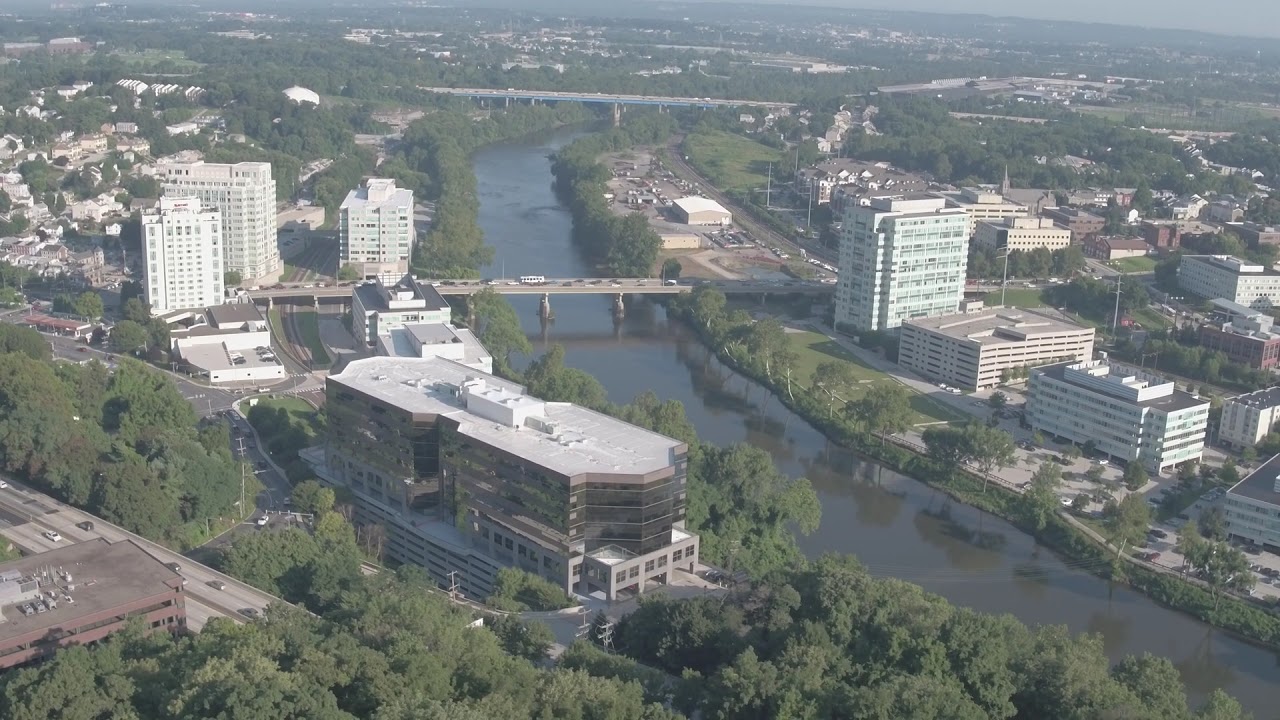This drone-shot image captures a far-out, daytime view of a city that strikes a balance between urban development and natural scenery. The cityscape features large, rectangular apartment buildings that reach up to 20 stories high, but it's not as dense as a typical metropolitan area like New York City. Divided by a dark blue and brown river, the city is connected by two bridges: one prominently stretching from the left to the right side of the image, and another in the distant background about half a mile away. The river flows diagonally from the lower right-hand corner and curves back to the right, framed by columns under the nearest bridge. Vehicles traverse the closest bridge, which is surrounded by clusters of treetops and foliage. The lower left of the image reveals a road snaking through this verdant canopy, contrasting with the sparser greenery and more visible parking lots on the opposite riverbank. A filmy haze adds a slightly off-colored gray tone to the picture, further enhancing the atmospheric quality of the scene. Prominent among the buildings is one that could possibly be a hospital, standing out due to its broad base and notable height.